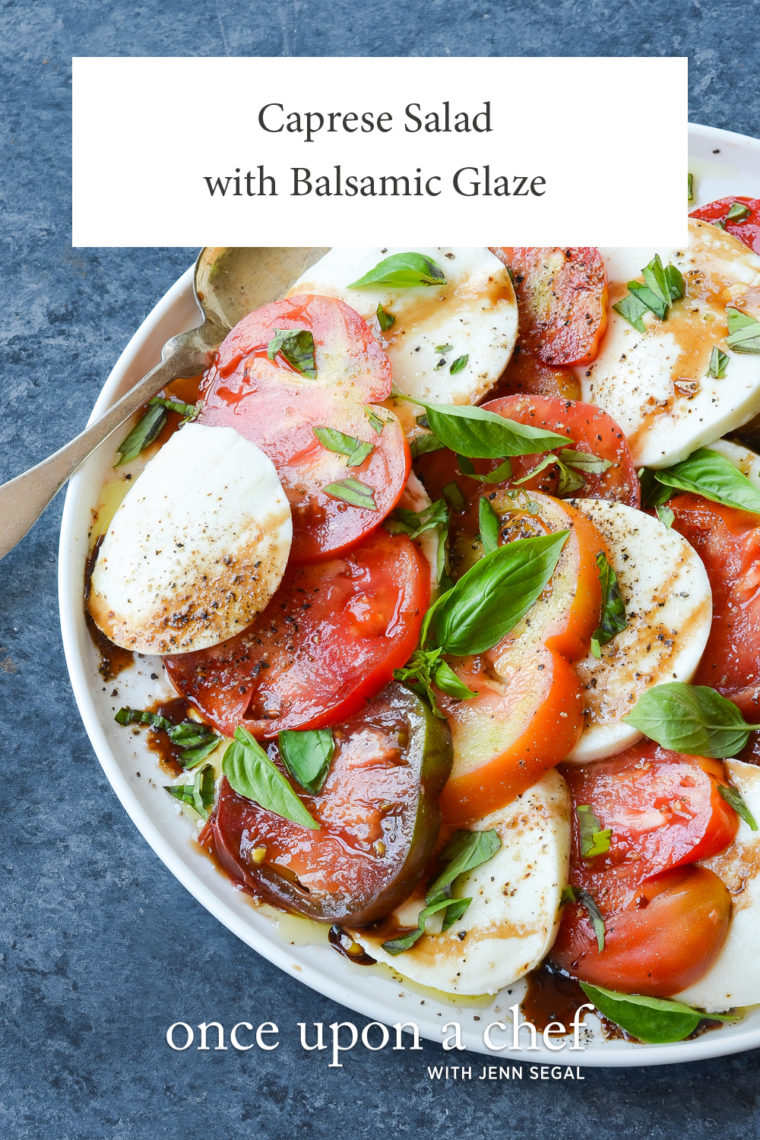The image features a white plate set against a dark blue background, presenting a Caprese Salad with Balsamic Glaze. At the top of the image, bold dark letters on a white background read "Caprice Salad with Balsamic Glaze," while the bottom right corner displays the text "Once Upon a Chef with Jen Siegel." The salad is arranged with alternating thin slices of juicy, round tomatoes and fresh mozzarella cheese that are nearly uniform in size. Scattered throughout the salad are vibrant basil leaves, adding a touch of green. A fork is positioned from the left center edge of the plate, ready to dive in. The dish is elegantly drizzled with a dark brown balsamic glaze, creating delicate stripes over the tomatoes, mozzarella, and basil, enhancing the visual and flavor appeal without overwhelming the ingredients.